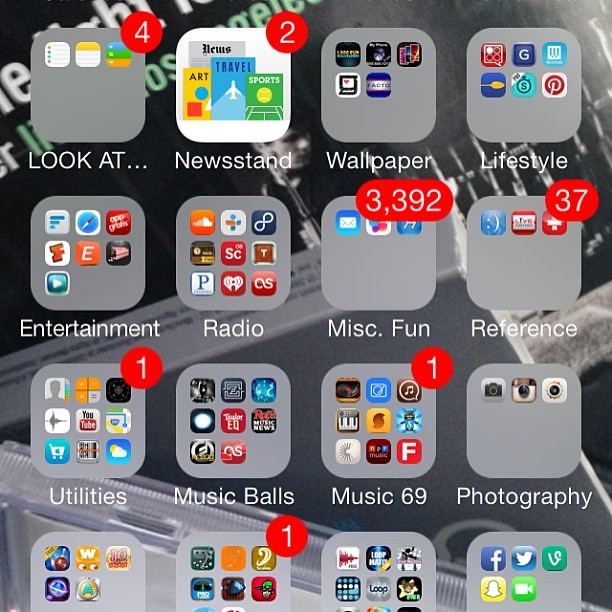This image is a close-up screenshot of a smartphone display, with the typical top and bottom information bars obscured. The background features a gray and black aesthetic with what appears to be CD cases or music covers behind the app icons. At the center of the background is a man standing next to a microphone. The layout comprises four rows and columns of app folders.

**First Row:**
1. **Top Left Folder**: Gray square with three smaller squares inside, labeled "Look at..." in white. A red circle with the number 4 is in the top-right corner.
2. **Second Folder**: White circle containing four magazine-like icons (short yellow, tall blue, short green, and a white one behind them), labeled "News Stand."
3. **Third Folder**: Gray, containing five smaller icons, labeled "Wallpaper."
4. **Fourth Folder**: Gray with six icons, labeled "Lifestyle."

**Second Row:**
1. **First Folder**: Contains seven smaller icons, labeled "Entertainment."
2. **Second Folder**: Contains nine smaller icons, labeled "Radio."
3. **Third Folder**: Features three smaller icons, and a red circle with "3392" in white letters at the top-right corner, labeled "Miscellaneous Fun."
4. **Fourth Folder**: Contains nine icons, a red circle with "1" in it, labeled "Utilities."

**Third Row:**
1. **First Folder**: Contains eight icons, labeled "Music Balls."
2. **Second Folder**: Contains nine icons with a red circle and "1" in it, labeled "Music 99."
3. **Third Folder**: Contains three icons, labeled "Photography."

**Fourth Row (Partially Visible):**
1. **First Folder**: Contains five icons (label not visible).
2. **Second Folder**: Contains eight icons, with a red circle and "1" in it.
3. **Third Folder**: Contains nine icons.
4. **Fourth Folder**: Contains five icons.

The overall composition of the screenshot highlights a structured arrangement of various app categories. Each folder is neatly labeled, providing insight into the thematic organization of the smartphone's home screen.